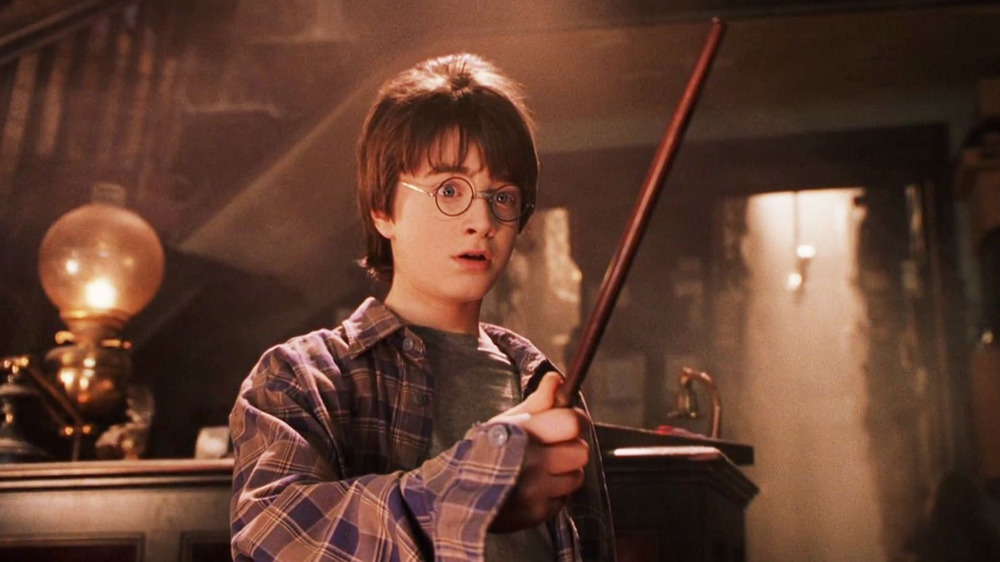The image depicts a young boy, easily recognizable as Harry Potter from the movie series. He is positioned slightly left of center in the horizontal, rectangular frame. Harry is wearing circular wireframe glasses and has medium-length brown hair with bangs in front. His expression appears scared or mystified, with his mouth slightly open. He is dressed in a blue and brown checkered long-sleeve plaid shirt over a gray t-shirt. 

In his extended right hand, slightly in front of his body and closer to the bottom middle of the picture, he holds a brown wand that extends upward and to the right, almost reaching the top of the frame. The boy is cut off at the midsection by the bottom of the photo. 

The background is dimly lit, suggesting an old, somewhat mysterious setting. To his left, a kerosene lamp sits on a dark-colored wooden table, which also holds some indistinguishable items. Behind the table, a staircase with a railing is visible, and to Harry's right, there's a doorway leading to another room with light streaming through. The overall focus remains on Harry Potter, capturing a moment of surprise or shock.